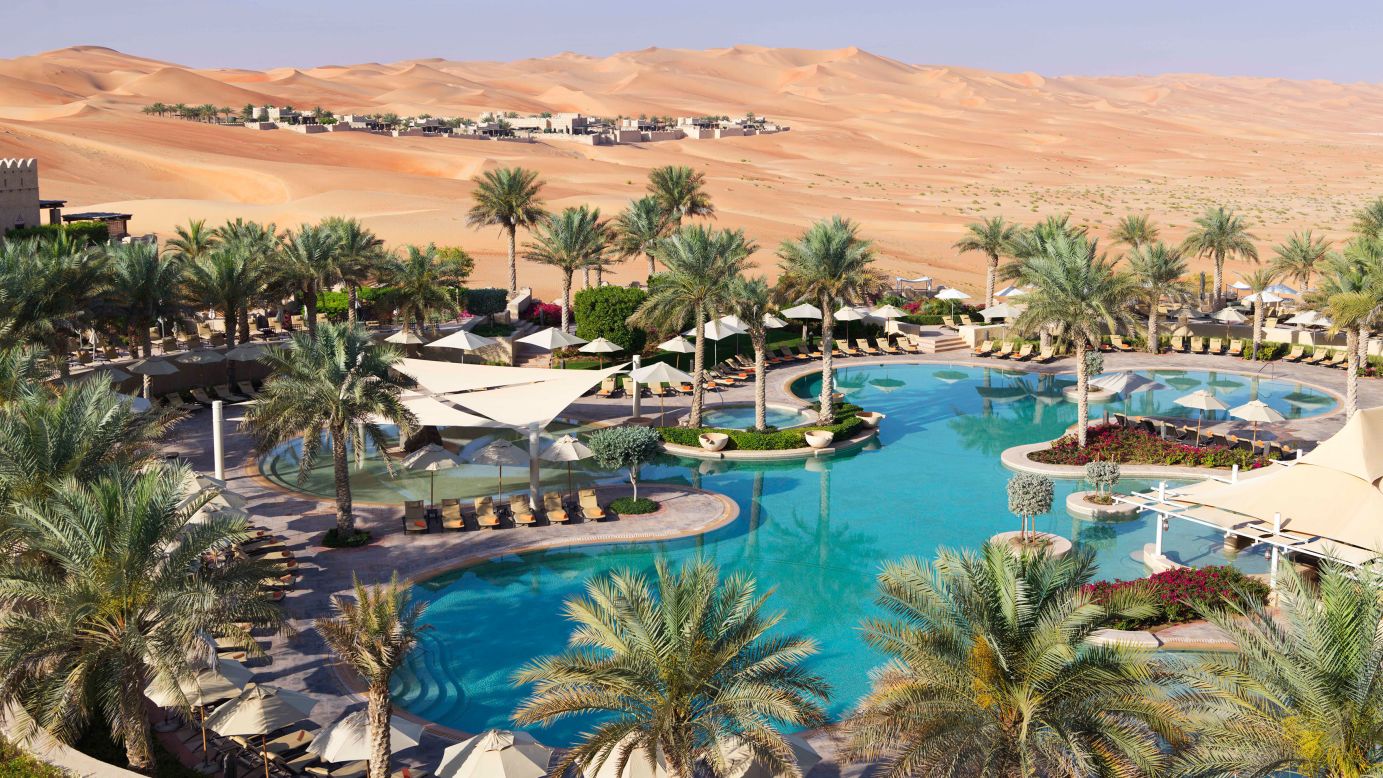This professionally captured image showcases a stunning resort oasis situated in the heart of a barren desert landscape with hills shaped by winds. The focal point is a large, uniquely shaped pool resembling a flower with rounded, sculpted edges filled with greenish-blue water. Surrounding the pool are numerous deck chairs and white shade umbrellas, along with an abundance of tropical palm trees and scattered red flowers, providing an inviting contrast to the arid backdrop. In the background, a small town with predominantly white and tan buildings is visible, with one particularly notable structure featuring castle-like architecture partially obscured by the verdant trees. The scene suggests that water must be imported to sustain the lush greenery and fill the pool, emphasizing the resort's separation from its natural desert surroundings.